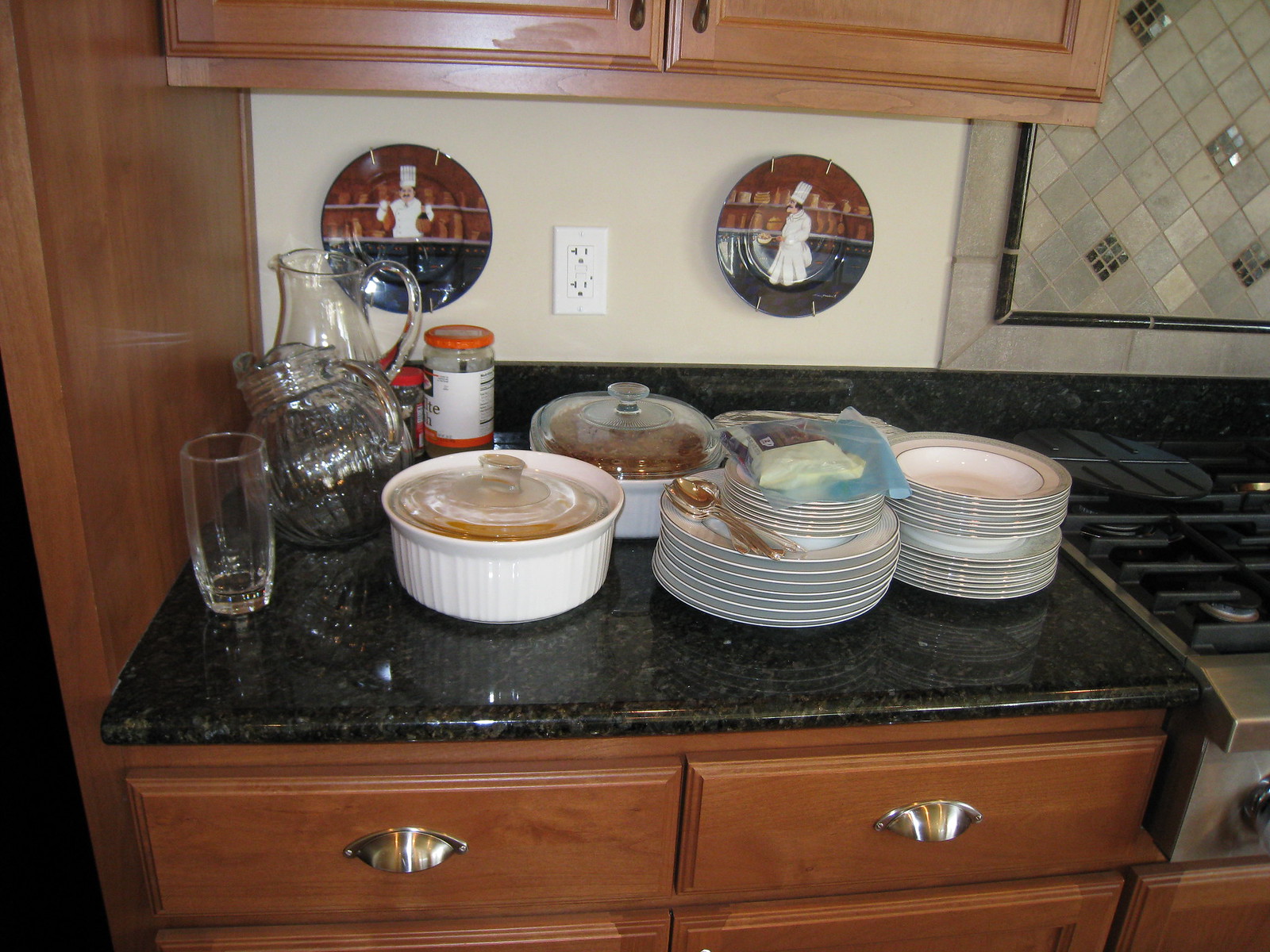The image showcases a well-organized kitchen counter, highlighting its black marble surface that elegantly contrasts with the wooden drawers beneath. Above the counter, wooden cabinets align perfectly with the aesthetic, complementing the overall warmth of the setting. The backdrop is a pristine white wall, adorned with two decorative plates and an electrical outlet neatly centered.

The countertop is actively in use, with several stacks of dinnerware arranged meticulously. Multiple plates, saucers, and bowls are piled up, ready for their next use. On the left side of these stacks, two white CorningWare bowls with clear lids, containing some food, sit prominently. Further to the left, a pair of large glass pitchers with visible handles and tops are positioned near the wall, accompanied by a single drinking glass placed in front of them.

Adjacent to these items, on the right side of the counter, a black gas stove with sturdy black grates comes into view, suggesting a functional and frequently-used kitchen space. The overall arrangement beautifully illustrates both the practicality and aesthetic appeal of this culinary corner.